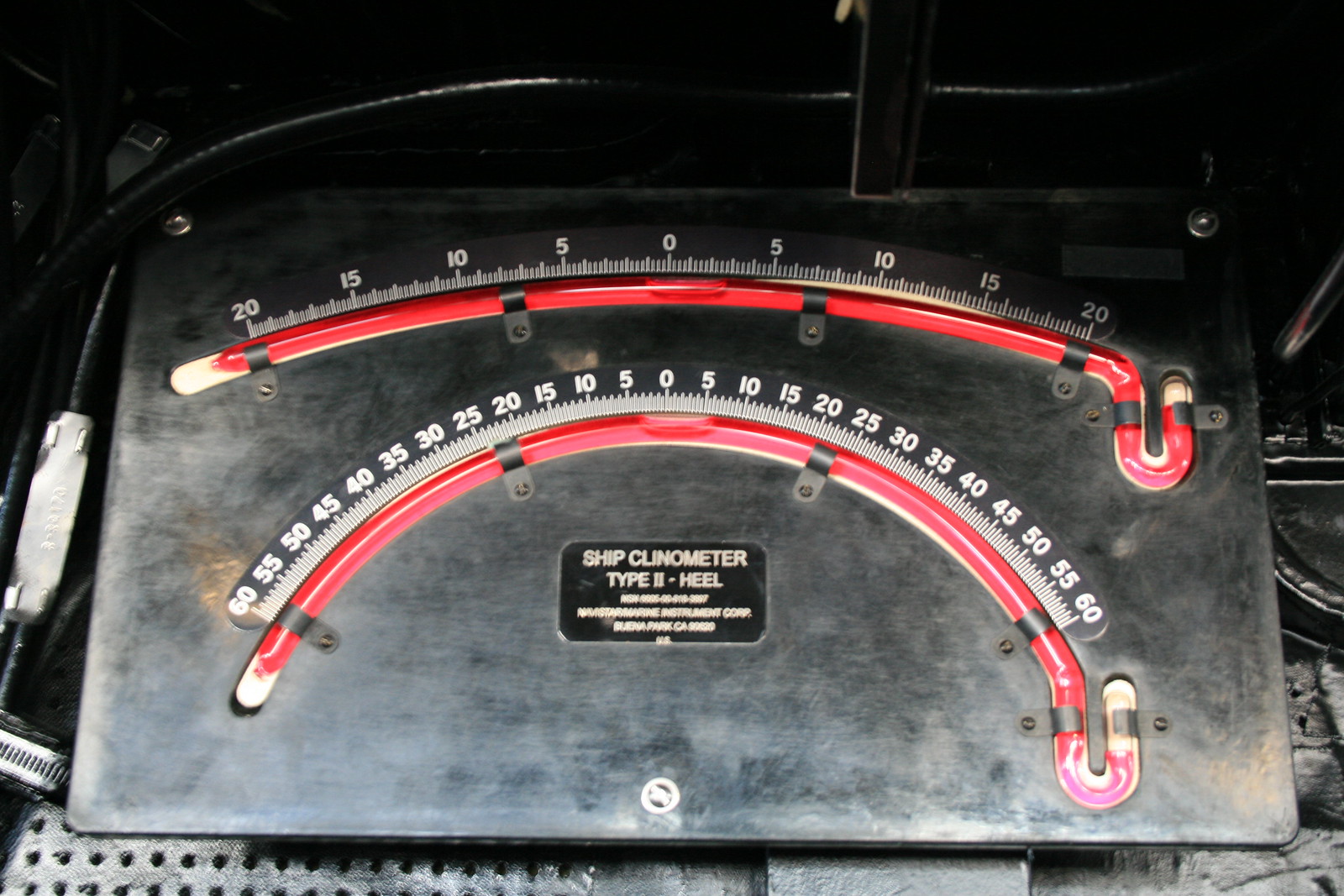The image showcases a detailed display featuring a SHIP Clinometer Type II, labeled clearly in the center with "HEAL." This precision instrument includes two prominent gauges with red indicators, and strategically placed numbers in white for clear readability. 

The top gauge, a horizontal linear meter, spans from -20 to 20 with increments of 5, centering at zero. Below it, situated centrally, is a curved arc meter, extending from -60 to 60, also marked in increments of 5 and having its midpoint at zero. Both gauges are encased within a sturdy black framework, securely fastened with strategically positioned black straps. Four straps anchor these meters at symmetrical points, while a fifth strap extends from the right side, featuring a distinctive U-shaped clasp that stretches upward toward the top meter.

Each gauge contains red liquid, which appears to be a crucial component for measurement. The entire assembly, primarily black, is visibly positioned in the zoomed-in portion of a car trunk, suggesting a portable or transportable setup for precise inclination measurements.